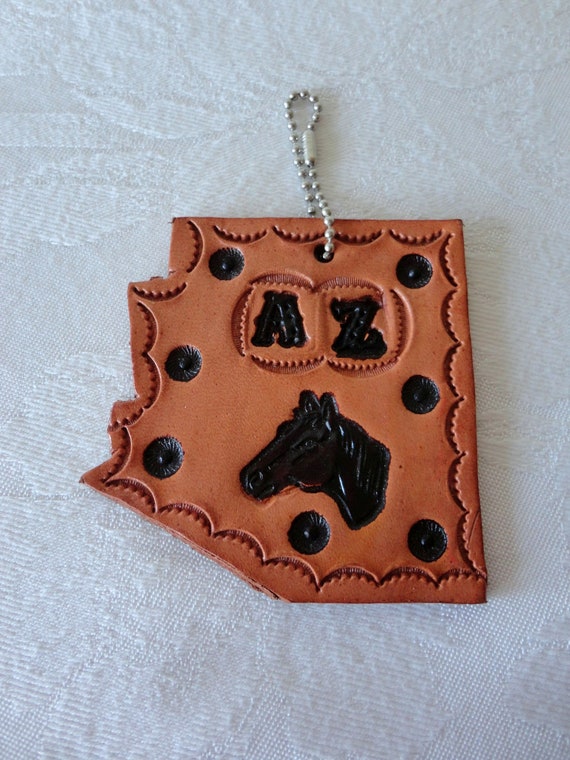The vertically aligned rectangular image features a brown leather keychain placed on a subtly patterned white textured tablecloth. The tablecloth's design hints at either a leaf or floral motif. The keychain, shaped reminiscently of the state of Arizona, features multiple intricate design details. Its leather is bordered by black circles and an outer arc of eyelash-like shapes shaded in black. Near the bottom center, a black embossed horse's head is prominently displayed, while initials, likely A and Z, are positioned just above it. The keychain, detailed with half-moon and other indentations, has a cut-out at the top attached to a small silver clasp chain, perfect for holding keys.